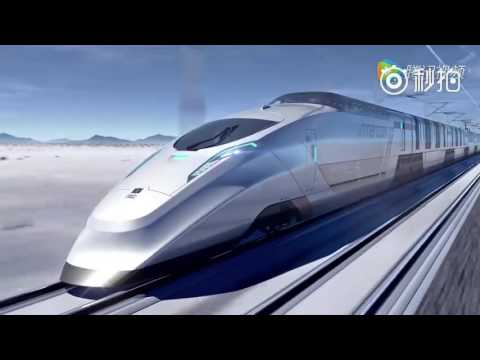The image showcases a sleek, high-speed bullet train, likely a computer-generated concept. With a modern, silver and white exterior accentuated by turquoise-green glowing lights at the very sloped front, the train exudes a futuristic allure. A black front window, presumably for the control room, and a series of side windows and panels, possibly for luggage, adorn the streamlined body. The train travels on an elevated, white and gray track set on a gray brick overpass, slicing through a deserted, white sandy landscape. The background reveals sparse vegetation and low, bluish-gray mountains against a light blue to silvery-gray sky. In the upper right corner of the image, Asian script accompanies a bullseye symbol, adding an element of cultural intrigue.